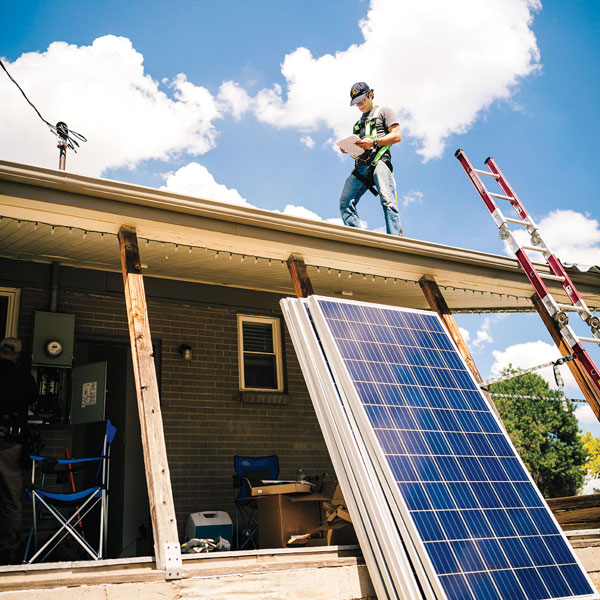This image captures a daytime scene of a single-family home construction site. Prominently, a white man stands on a porch roof, wearing a gray shirt, blue overalls, and a blue hat, along with a green vest. He's engrossed in reading a piece of paper, possibly installation instructions for solar panels, which are stacked nearby against the house. The house itself features dark-colored brick with a small bathroom window visible beneath the porch awning. Next to the man, a red and white ladder leans against the roof. Below, the porch area under the overhang is cluttered with various construction tools, a blue and white cooler, two blue foldable chairs, and a blue lunch pail. There are also green breaker boxes attached to the side of the house. The wooden beams supporting the porch overhang seem newly reinforced, although the porch appears to need a fresh coat of paint. Christmas lights are strung along the awning, adding a festive touch to the scene. In the background, a blue sky peppered with fluffy white clouds suggests a sunny day, highlighting the overall sense of construction activity and progress.